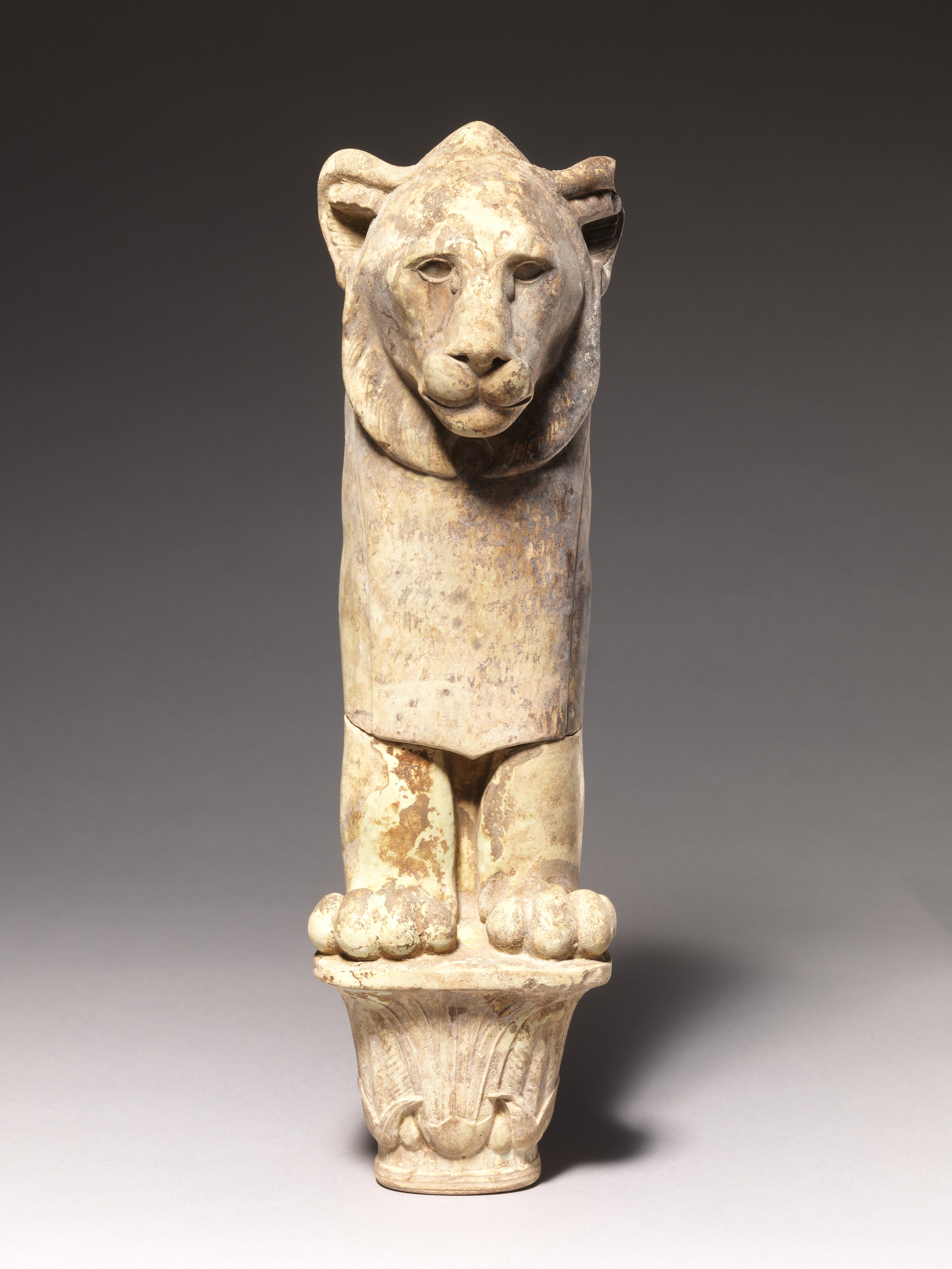The image features an aged statue of a lion, meticulously crafted from tan or white marble, with evident signs of wear. The lion stands majestically on a decorative podium, staring ahead with a dignified expression, its features including the eyes, nose, and mouth clearly discernible. The lion's sculpted mane cascades down its neck, and both ears are visible, although the right ear is slightly damaged, indicating the statue's age. The front paws of the lion are detailed, with four fingers on the left paw and three visible on the right paw. The backdrop is a simple white room, accented by gray shades that enhance the statue's shadow, emphasizing its presence.